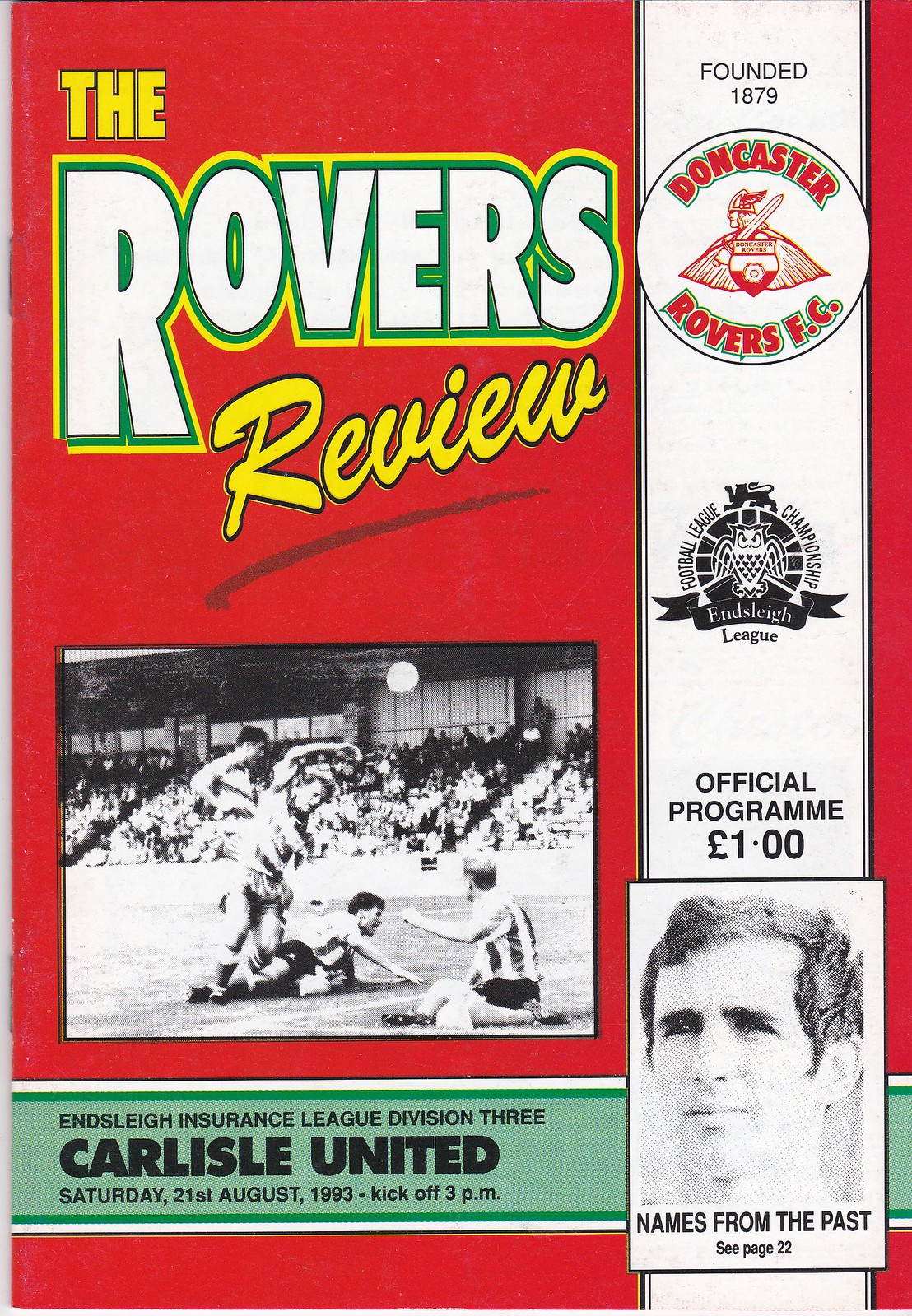The image appears to be the front cover of a program flyer titled "The Rovers Review," primarily red with white and yellow text. "The Rovers" is prominently displayed with "The" in yellow and "Rovers" in white, followed by "Review" in yellow text. A vertical white bar runs along the right-hand side, with text noting "Founded 1879" and a small circular logo detailing "Doncaster Rovers F.C." in red. The cover features a black and white photograph of a soccer match where players and a referee are visible, suggesting a dynamic in-game moment with the soccer ball in mid-air. Additionally, a smaller black and white photo of a soccer player is labeled "Names from the Past, see page 22."

In the top right, a knight with a cape and sword symbolizes the team's logo, reaffirming "Doncaster Rovers F.C." and the establishment date. The program is referenced as the "Official Program" costing one dollar or euro. Information about the match "Enslay Insurance League Division III, Carlisle United," dated "Saturday, 21st of August, 1993, kick-off 3 p.m." appears in a green footer. It's a detailed snapshot of the Doncaster Rovers' soccer team program from 1993.